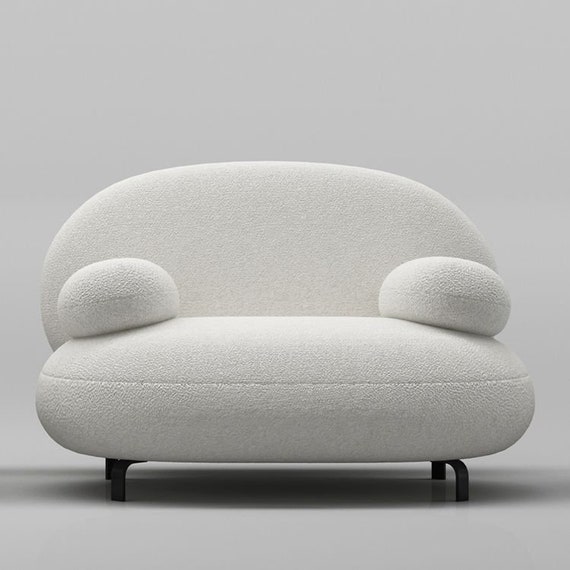This photograph captures a modern, eye-catching piece of furniture that blurs the line between a large chair and a small sofa. The design is characterized by its unique, very rounded features, giving it an elliptical silhouette. The backrest is a completely oval cushion, seamlessly mounted on the base, which is also oval-shaped. The armrests, resembling squished bowls or circular pillows, attach to each side, further emphasizing its unconventional look. 

Upholstered in an off-white, almost cream color, the fabric appears fuzzy, adding a tactile quality to its visual appeal. The piece sits on four short, dark metal legs, around five inches tall, providing slight elevation from the light gray floor. Set against a similarly light gray background, this stylish loveseat or chair stands out due to its artsy and minimalist aesthetic, making it more of an artistic statement than a practical seating option.